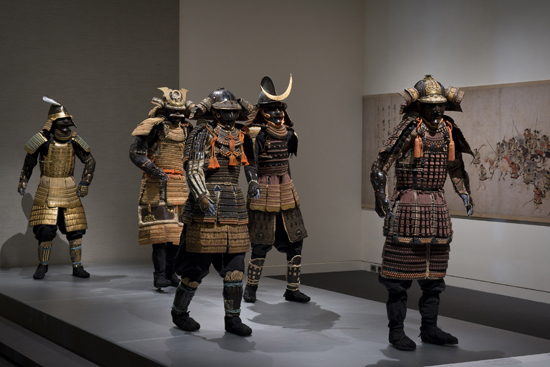The photograph, a full-color image taken indoors with artificial lighting, captures a detailed museum exhibit of samurai warriors in full regalia. The square image, devoid of any distinctive border, showcases five mannequins dressed in traditional samurai armor, standing on a slightly raised gray tile platform. The warriors' armor exhibits a range of colors from gold and brown to tan and purplish hues, complemented by intricate black and gold boots. Each warrior dons a unique helmet; one features a large crescent moon shape, while others have varying designs, including a round helmet with gold trim. Their armor includes elaborate shoulder pads, armored skirts, and leather gloves, adding to their imposing presence. The group formation has one warrior at the forefront, slightly to the right, leading four others who follow in a staggered arrangement. The backdrop includes light brown walls with a large horizontal painting on the right, possibly depicting flowers or fruit, adding to the museum-like ambiance. The detailed setup and the ornate costumes hint at a meticulously curated exhibit, aimed at showcasing the historical grandeur of samurai warriors.